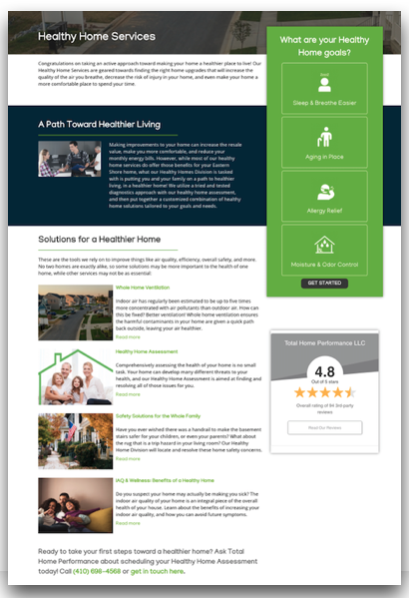Image Caption: The top left corner features a header that reads "Home Health Services," accompanied by some small, unreadable text on a white background. Directly below is a blue banner with the phrase, "A Path Towards Healthier Living." The central area includes a photograph, accompanied by a substantial paragraph of white text that is illegible. Beneath this section, there is a white background extending to the bottom of the image, topped with the phrase, "Solutions for a Healthier Home," highlighted by a green dividing line. Below the line is a black-text paragraph that is not readable. Adjacent to this, on the left side, is another photograph with some unreadable elements to its right. Four pictures are vertically aligned along the right-hand side. Each picture is accompanied by green headers and black informational text, all of which are unreadable. In the top right corner, a green vertical band encompasses four boxes, each labeled with text suggesting "sleep and breathe easier," "age in place," and "allergy relief," although it’s partially unreadable. The green band's title appears to be, "What Are Your Healthy Home Goals?" accompanied by white lines, icons, and text. At the bottom right corner, a rating of 4.8 stars is visible.